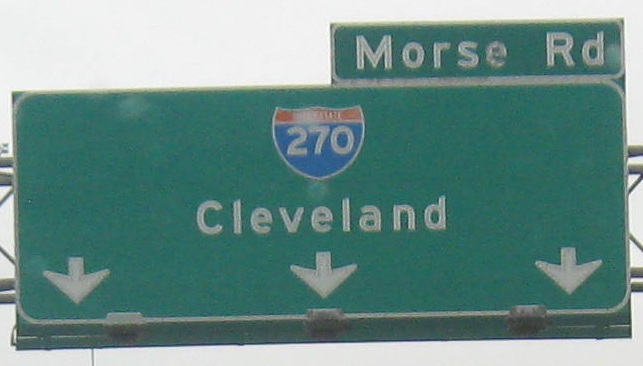The image depicts a highway sign supported by a large, 3D square-shaped metal brace that spans the entire width of the major highway. The metal framework in the background includes thick metal bars arranged in an X pattern, providing robust support for the signs. The signage itself is composed of two distinct elements, both solid forest green with white outlines.

On the smaller, rectangular sign, the text reads "Morse Road" with capitalized 'M' and 'R'. Adjacent to it is a much larger, wider sign which prominently displays a red and blue Interstate 270 emblem accompanied by the text "Cleveland". Below this, three arrows indicate the direction for drivers wishing to exit the highway to join Interstate 270 heading towards Cleveland.